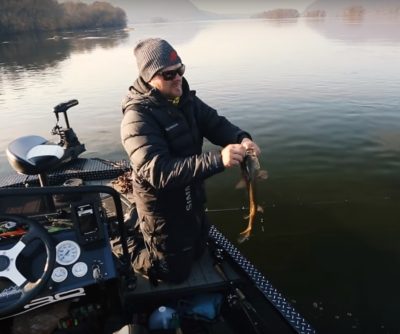In this image, a man is perched on a boat in the tranquil waters of a lake, surrounded by a serene and misty landscape. The water, characterized by gentle ripples and a brownish hue, extends across the scene, with the boat floating effortlessly. In the upper portion of the image, a sliver of cloudy sky can be seen, hinting at the cold, misty weather, along with the faint outlines of mountains or hills in the background. To the upper left, trees line the shore, adding a natural frame to the setting.

The man, bundled up against the cold, wears a gray beanie with an orange logo on the front, along with a heavy coat and sunglasses. His hands proudly hold a fish with a bright brown tail and a gray body, suggesting a recent catch. Although the fish is somewhat blurry, his pride is evident. The boat itself, mostly black on the inside, features a visible steering wheel and various round dials in the lower left corner. The scene captures a moment of quiet triumph in a picturesque, cold, and misty lakeside setting.